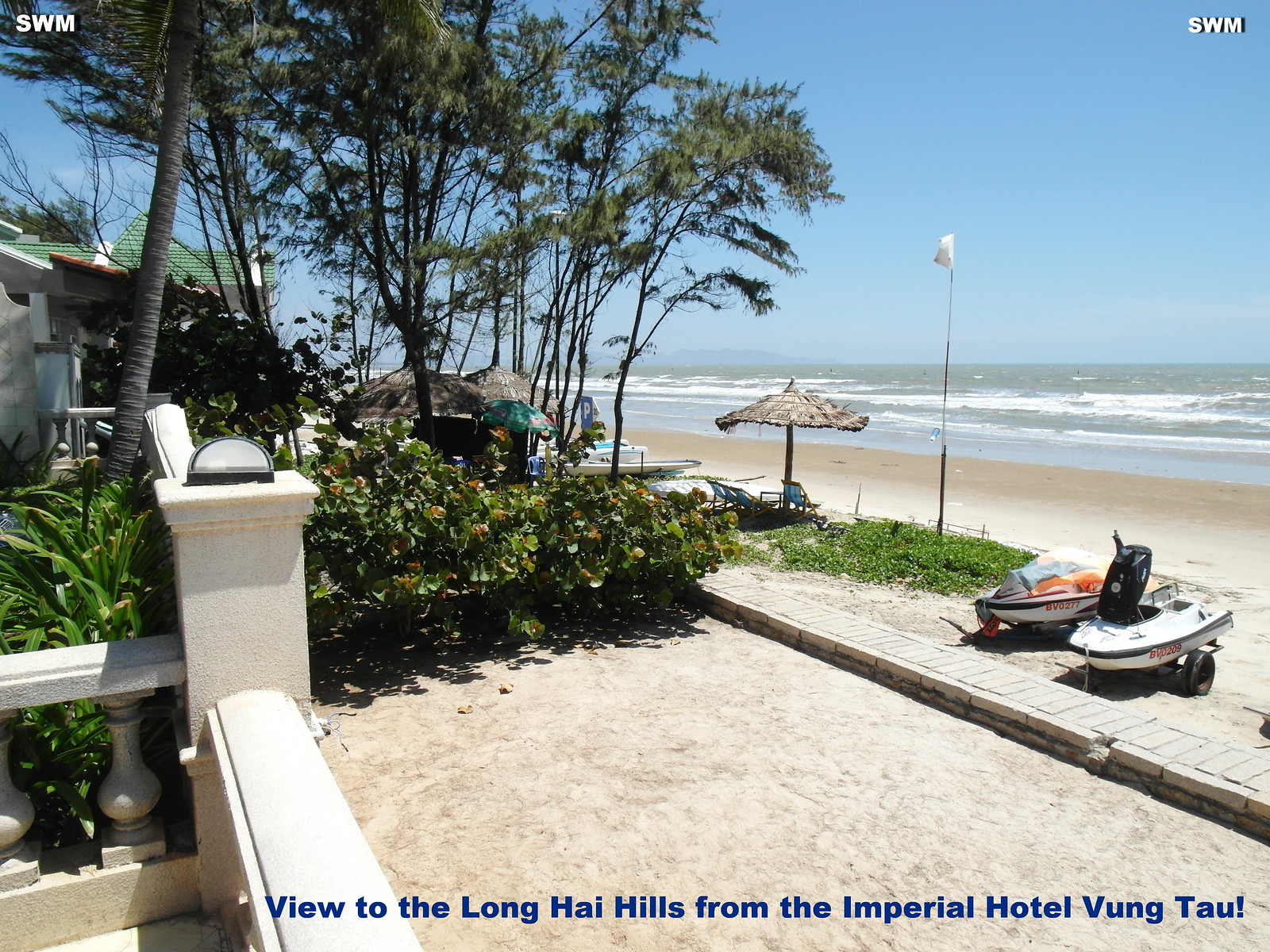This photograph captures a vibrant seaside scene, likely taken from a hotel room or a beach house, overlooking a beautiful stretch of coastline at the Imperial Hotel in Vung Tau. The foreground is dominated by a sandy beach where waves crash gently ashore, while a couple of boats are parked near a grassy patch beneath a beach umbrella accompanied by several chairs. A stone wall runs further inland, marking the boundary before revealing another sandy area dotted with shrubs. In the bottom left corner, a stone fence can be seen with a white-walled, green-roofed building situated beyond it, surrounded by trees. The clear blue sky suggests it is midday, adding an inviting glow to the expansive ocean view. In the distance, mountain ranges or islands rise majestically over the water. The image also features a caption in blue text at the bottom, stating, "View to the long high hills from the Imperial Hotel, Vung Tau," reinforcing the scenic beauty from this elevated vantage point.